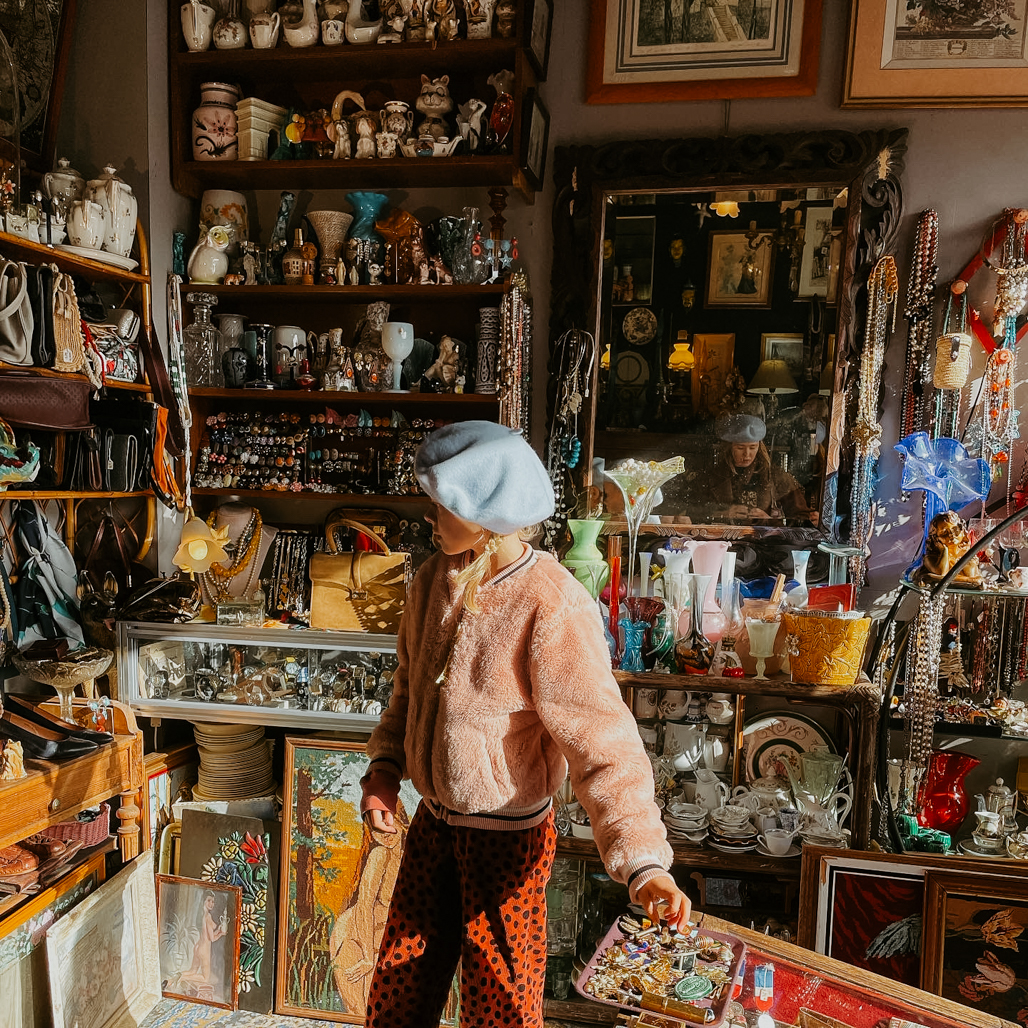The image depicts the interior of a dimly lit antique shop, brimming with a wide assortment of eclectic items. The shelves are crowded with a variety of vases, cups, saucers, and what might be stacks of plates. Among these items, numerous beads are scattered around, contributing to the store's cluttered ambiance. Two notable drawings or paintings are displayed, one of which features a naked woman by a tree. 

A white woman, possibly a young girl, is positioned to the left, examining the shelves. She wears a light blue beanie and a fuzzy pink jacket, paired with orange pants speckled with brown or gray spots. Her figure casts a shadow due to the uneven lighting. Behind her left shoulder, there is a striking light green vase, a color that notably stands out. 

In the center, an intriguing blue object catches the eye; its round and somewhat open shape suggests it could be a candle holder, complementing the store's apparent inventory of candles. An array of colors such as rust, light peach, orange, blue, red, black, white, gray, pink, yellow, and various shades of green pervade the scene, reminiscent of an artist’s palette. This vibrant color spectrum adds to the impression of a place filled with singular, mismatched treasures typical of an antique shop.